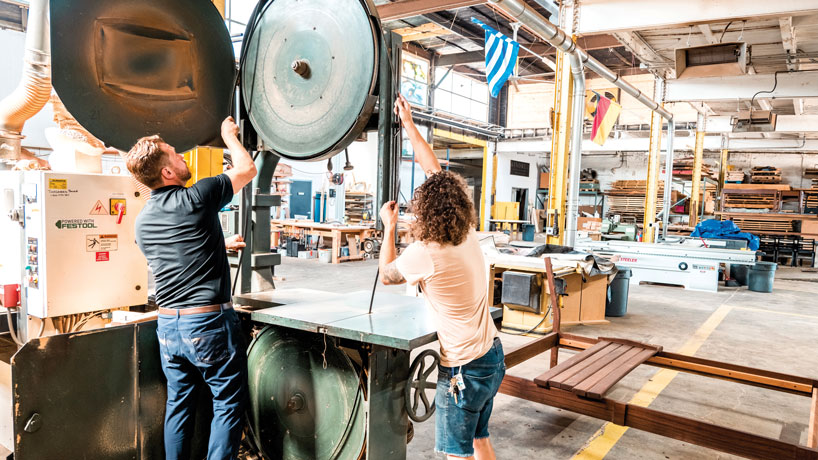The image captures the bustling interior of a well-lit manufacturing warehouse or workshop. Dominating the scene are a man and a woman engaged in a task involving a large, rust-colored metal wheel, suspended in the air. The wheel, with a central nut, appears to be part of a belt-driven mechanism, as both individuals pull on a black belt or cable from opposite sides. The man, with slicked-back dark brown hair and a beard, wears a black shirt, blue jeans with a brown belt. The woman, with curly dark brown hair, sports a beige shirt, blue jean shorts, and has a set of keys dangling from her pocket.

Surrounding them is an array of industrial components and equipment, highlighting the complexity of the workspace. The background reveals extensive shelving units loaded with dark wooden panels and bedposts, suggesting woodworking activities. A variety of machinery, including lathes and exhaust fans, populate the area, supported by high ceilings with I-beams painted yellow. Metal piping snakes across the ceiling, contributing to the mechanical ambiance.

The concrete floor, marked by distinct yellow lines, further solidifies the industrial setting. Additional elements include wooden pallets, boxes, and tables cluttering the space. Flags—one blue and white, the other yellow and red—hang overhead, adding splashes of color to the otherwise utilitarian scene. More tables and shelving units are seen in the distance, along with an open garage door featuring windows, offering a glimpse of the activity beyond the immediate foreground.